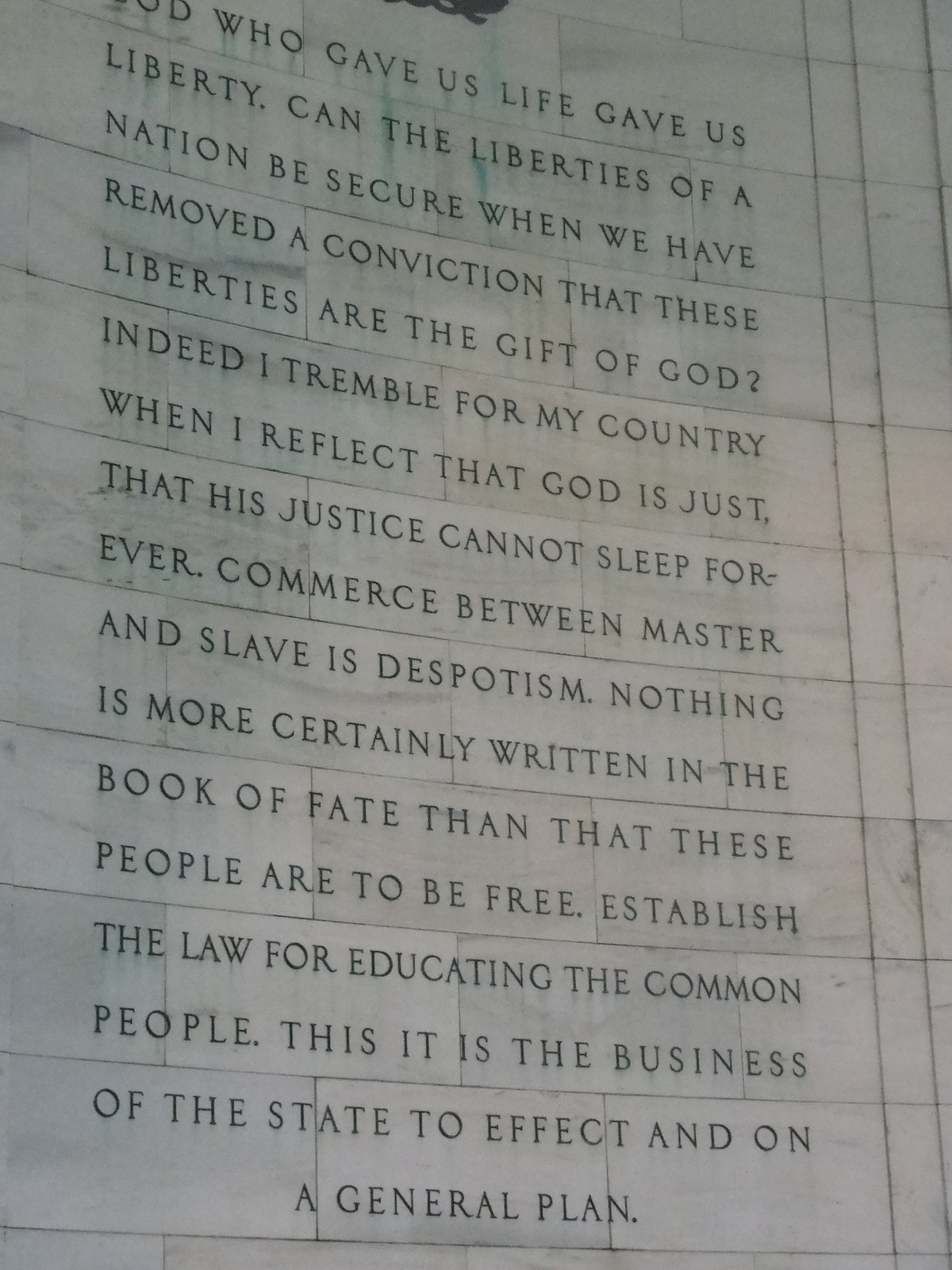The photograph, captured in portrait mode, presents a meticulously detailed image of a stone monument with an engraving. The monument is composed of light gray stone blocks, some large and some smaller, arranged in a concave bend. The surface exhibits horizontal lines and small rectangular bricks forming the structure of the façade. Etched onto this stone wall in black, all-capitalized text, is an inscription that reads: 

"God who gave us life gave us liberty. Can the liberties of a nation be secure when we have removed a conviction that these liberties are the gift of God? Indeed, I tremble for my country when I reflect that God is just, that his justice cannot sleep forever. Commerce between master and slave is despotism. Nothing is more certainly written in the book of fate than that these people are to be free. Establish the law for educating the common people. This it is the business of the state to effect and on a general plan."

The clarity of the etched words against the light gray stone creates a striking contrast, enhancing the solemn and reflective nature of the inscription, which appears to be a tribute or memorial.